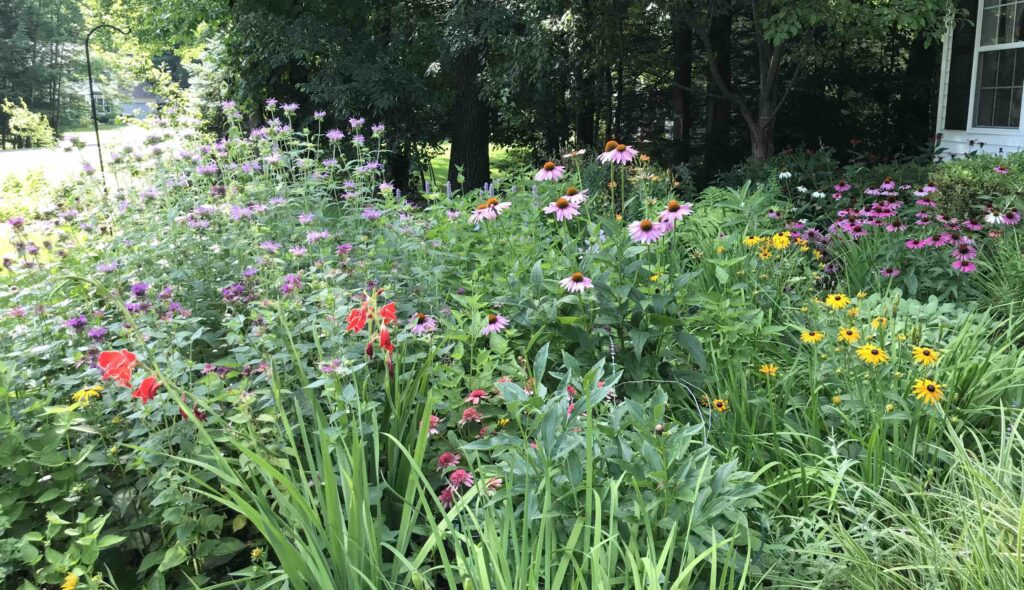A dense, overgrown garden sprawls in front of a white house with a black shuttered window visible in the upper right corner. The garden is a vibrant riot of colors, with various wildflowers including tall pink daisies, tiny reddish-pink blossoms, yellow flowers, and scattered dark purple and white blooms. These flowers intermingle without clear separation, creating a lush, haphazard display of nature’s abundance. Tall, leafy plants and sawgrass weave through the flower beds, giving the garden a wild and untamed appearance. In the background, tall trees with thick, green canopies tower over the scene, adding to the fullness of the backyard. Beyond the trees, there is a well-lit path or street, and possibly a vehicle, indicating a peaceful neighborhood setting.